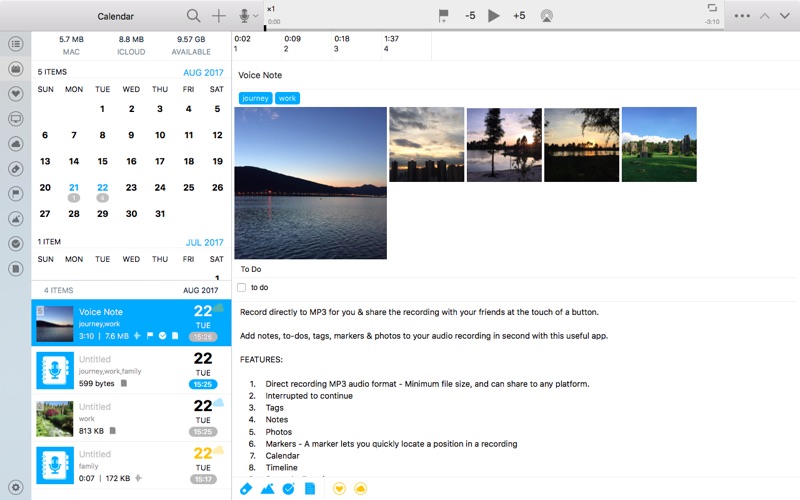The image is a detailed screenshot of a calendar interface, prominently displaying the month of August 2017 on the top left. Accompanying the calendar are five small beach-themed photos arranged just below it, adding a summery vibe to the visual. Underneath these pictures, textual information highlights the capabilities of an app, stating: "Record directly to MP3 and share the recording with your friends at the touch of a button." Further below, it explains additional features: "Add notes, to-dos, tags, markers, and photos to your audio recording in seconds with this useful app." The screenshot portrays both a functional calendar and a multi-featured recording app interface.